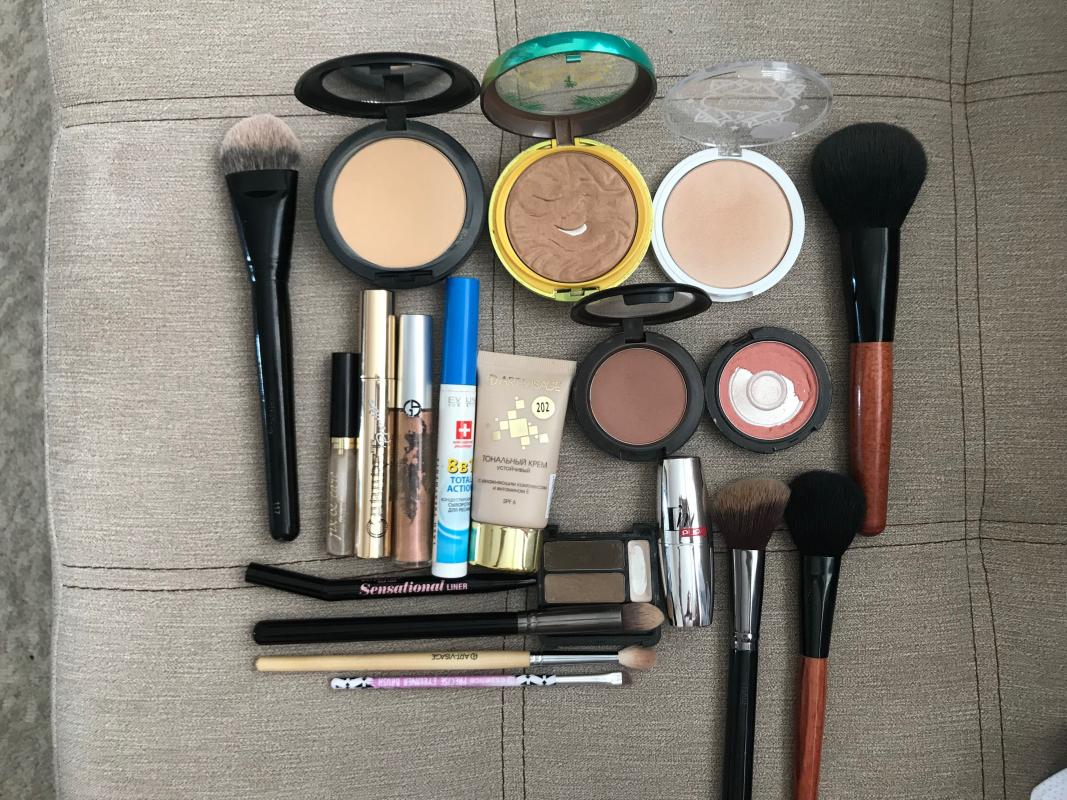The overhead image captures an extensive array of makeup and beauty tools meticulously spread across a brown surface. From the left-center, a long black-handled brush, which could be either a blush or foundation brush, dominates the view with its brown-tipped bristles. Adjacent to it lie three open powder compacts, each showcasing a gradient of brown powders. The central compact appears to house a darker bronzer, while nearby, a thicker black makeup brush stands poised for use.

In the middle row, several tubes presumably containing lip glosses catch the eye, featuring pink hues alongside one accented with gold. A small tube of foundation—recognizable by its gold-twist cap—adds to the collection, situated next to another compact holding a deep pink mocha shade of blush. Nearby, a half-used blush pot nestles among more beauty tools. Positioned beneath, a pair of additional makeup brushes appear ready for precise application.

To the left, a collection of slender makeup brushes, likely intended for eyeshadow or eyeliner application, extends to the far end, where a distinct pink and silver brush with short brown bristles is located. A sleek silver tube of mascara is strategically placed among the assortment of brushes, completing the comprehensive display of essential makeup items.